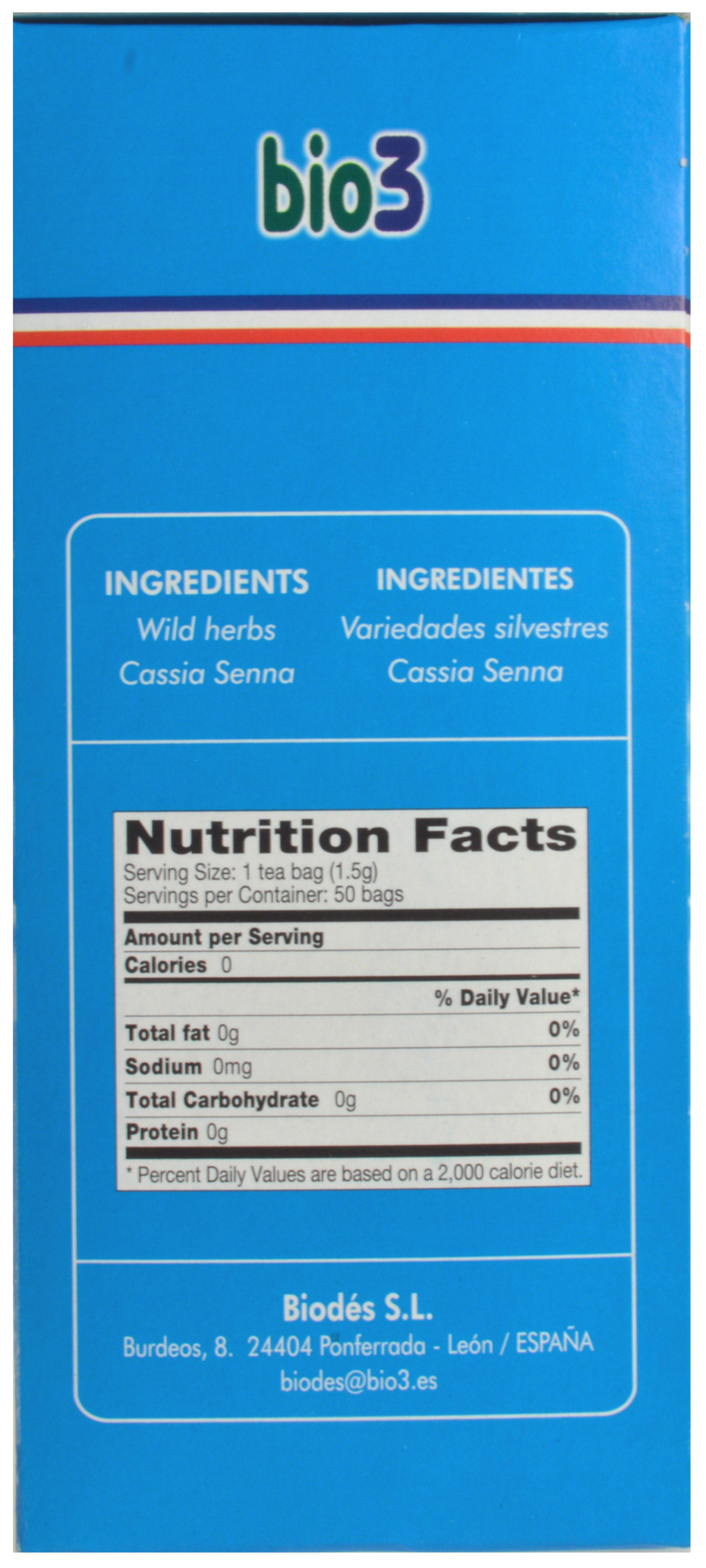The image showcases a vibrant, medium blue box, likely containing a food product such as tea bags. Dominating the top section, in green lowercase letters, is the word "bio," followed by a numeral "3" in navy blue, indicative of the brand, Bio 3. Complementing this branding, a tricolor stripe with blue, white, and red bands runs horizontally across the box.

Beneath this stripe, enclosed in a thin white-trimmed rectangular box, the word "Ingredients" is prominently displayed. Listed are "Wild Herbs" and "Cassia Senna," provided in both English and another language, potentially Spanish, as seen with "ingredientes" and "hierbas silvestres." 

The central part of the box transitions to the nutrition facts panel, presented in black print. It denotes serving details, specifying one tea bag per serving with 50 bags per container. Nutritional values highlighted include zero calories, total fat, sodium, total carbohydrates, and protein, affirming the nutritional simplicity of the product. 

At the bottom of the box, details about the manufacturer are spelled out: "Biodes S.L., Berdeo's 24 404 Ponferrada, León, España," alongside their website, "biodis@bio3.es."